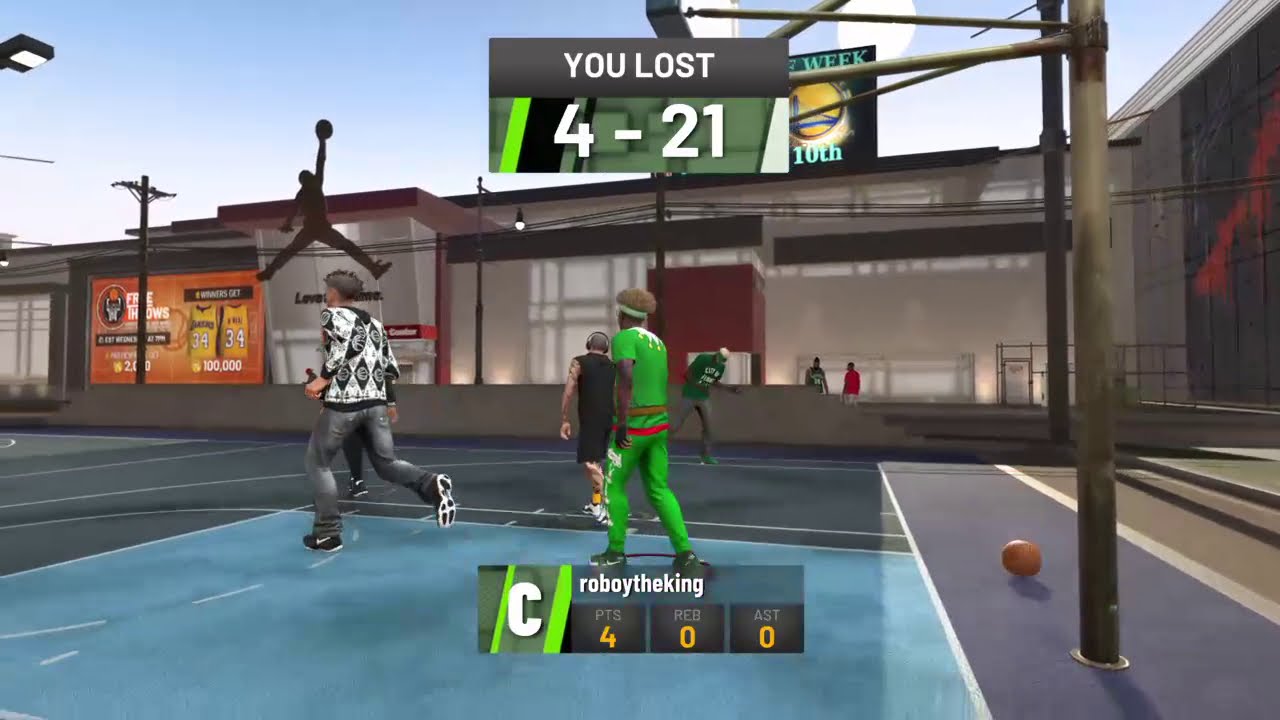This image is a detailed screenshot from a video game depicting a lively basketball game set in an outdoor courtyard among colorful, cartoonish buildings. The top of the image features a bright blue sky with a hint of cloudy haziness and a backdrop of one-story buildings lined with power poles and black power lines. A prominent yellow and orange advertisement sign featuring two yellow basketball jerseys with the number 34 can be seen on one of the buildings.

In the center of the image stands an African-American man in a green basketball outfit, marked with an orange line above the hips and a red line encircling his waist. A basketball is positioned on the right of this player, who is preparing to make a play. Adjacent to him, a man dressed in black and white long-sleeved outerwear, faded black jeans, and Nike tennis shoes is running away. Another African-American player in a green jumpsuit faces away from the camera, flanked by a Caucasian player with headphones, wearing a black tank top and shorts.

Further details include a rectangular sign near a basketball hoop on the right, which reads "You lost" in white lettering on a black stripe, followed by the score "4 to 21". Below this, the court's surface features square blocks of blue, gray, and dark green colors. The screen's bottom part displays the stats: "Roboy the King," four points, zero rebounds, and zero assists (AST). Additionally, there is a random Michael Jordan Air Jordan image hovering in the sky. The overall vibrant and dynamic setting captures the essence of an engaging basketball game.